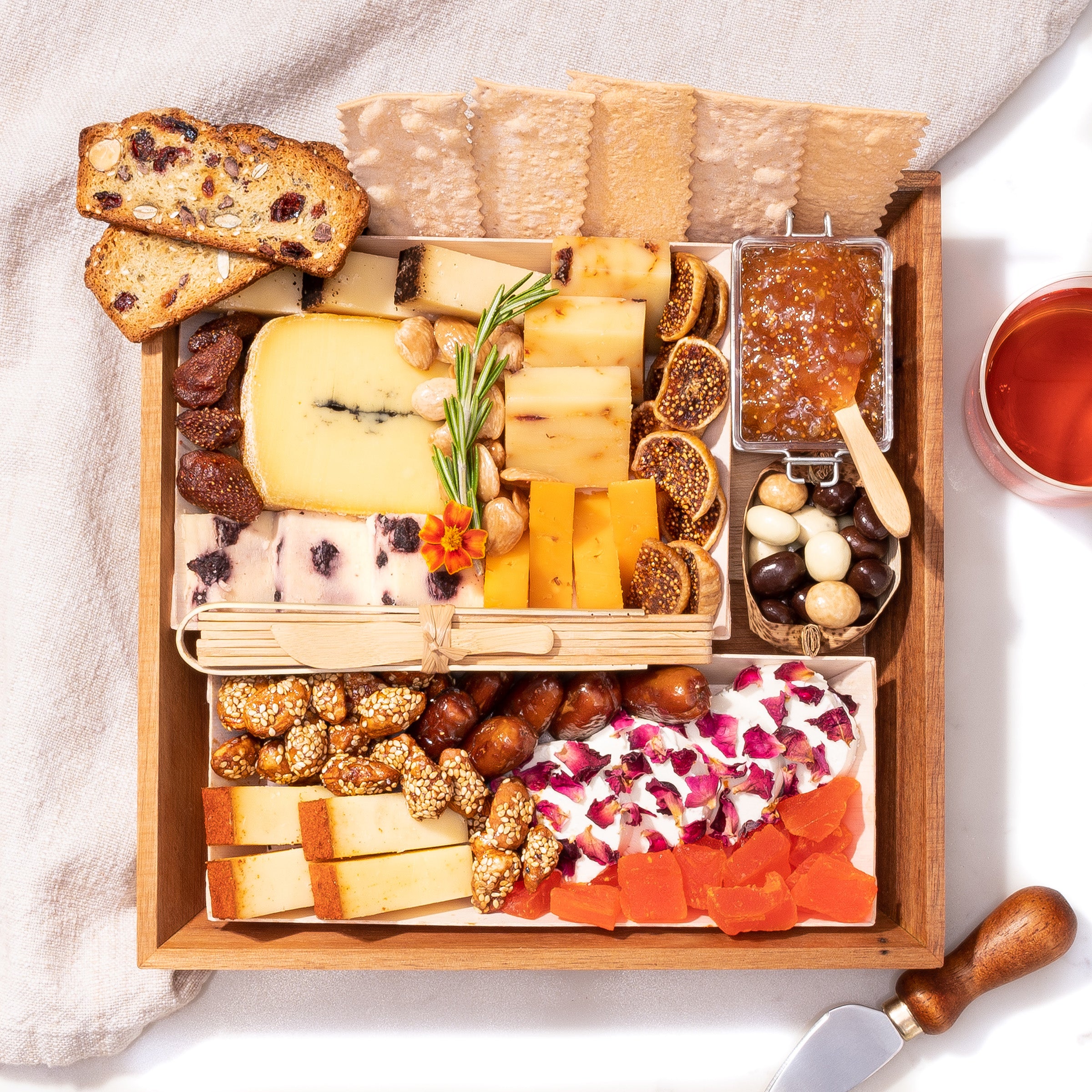The image depicts a well-appointed charcuterie board arranged within a square, three-dimensional wooden tray with a rich, finished hardwood appearance. This tray is partially resting on a cloth that's folded into a triangle and characterized by tan and white stripes. 

Starting from the top left of the tray, there are two slices of a raisin nut cake with visible fruit and nuts. To their right, several rustic-looking crackers lie next to five strips of dough, cooked to a white and tan color. Just below this section, a smaller rectangular white dish holds a variety of fruits and cheeses, including off-white, tan, and orange-colored cheeses, and a central sprig of greenery adorned with an orange flower.

Adjacent to this dish on the right is a container of what looks like apricot jam or marmalade, distinguished by its orange hue. Below this spread are yogurt or chocolate-covered nuts. Continuing downwards, at the bottom of the tray, there are artisanal brown pastries embellished with sesame seeds, next to four slices of a cake with a brown top and off-white base. Two white pastries topped with red fruit pieces are also present.

The edges of the tray feature assorted breads and crackers, and there is a collection of wooden utensils, including a spreading knife, in a dedicated holder. To the right side of the tray, a glass container holds golden honey, and at the bottom right corner of the image, a knife with a brown wooden handle is visible. The meticulous assortment of items showcases a mix of flavors and textures, embodying an elaborate and inviting spread.